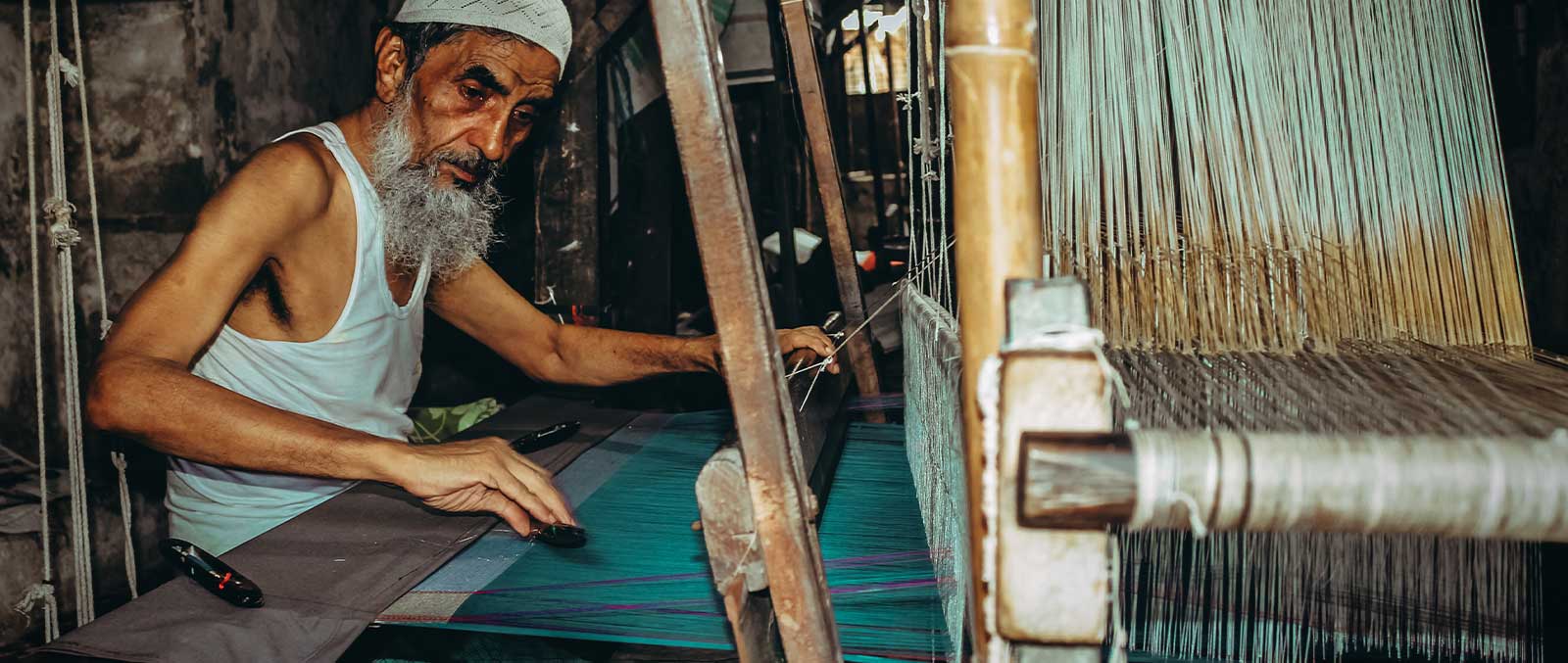The professional photograph captures an elderly, skinny man with a white-greyish beard and light brown skin, deeply engaged in working on an antique loom. Dressed in a white cap and a white undershirt, he sits at a wooden desk surrounded by countless strings attached to pulleys and levers. The loom holds a blend of white and brown threads, while the fabric he is meticulously weaving features intricate multicolored threads in shades of green, teal, and purple, appearing smooth and detailed. The setting, possibly in a rustic or Middle Eastern textile workshop, lacks natural light, with the scene illuminated primarily by the camera's flash. The man, who seems to be in his 70s but remains in good shape, focuses intently on crafting what could be a blanket, carpet, or another intricate textile product.